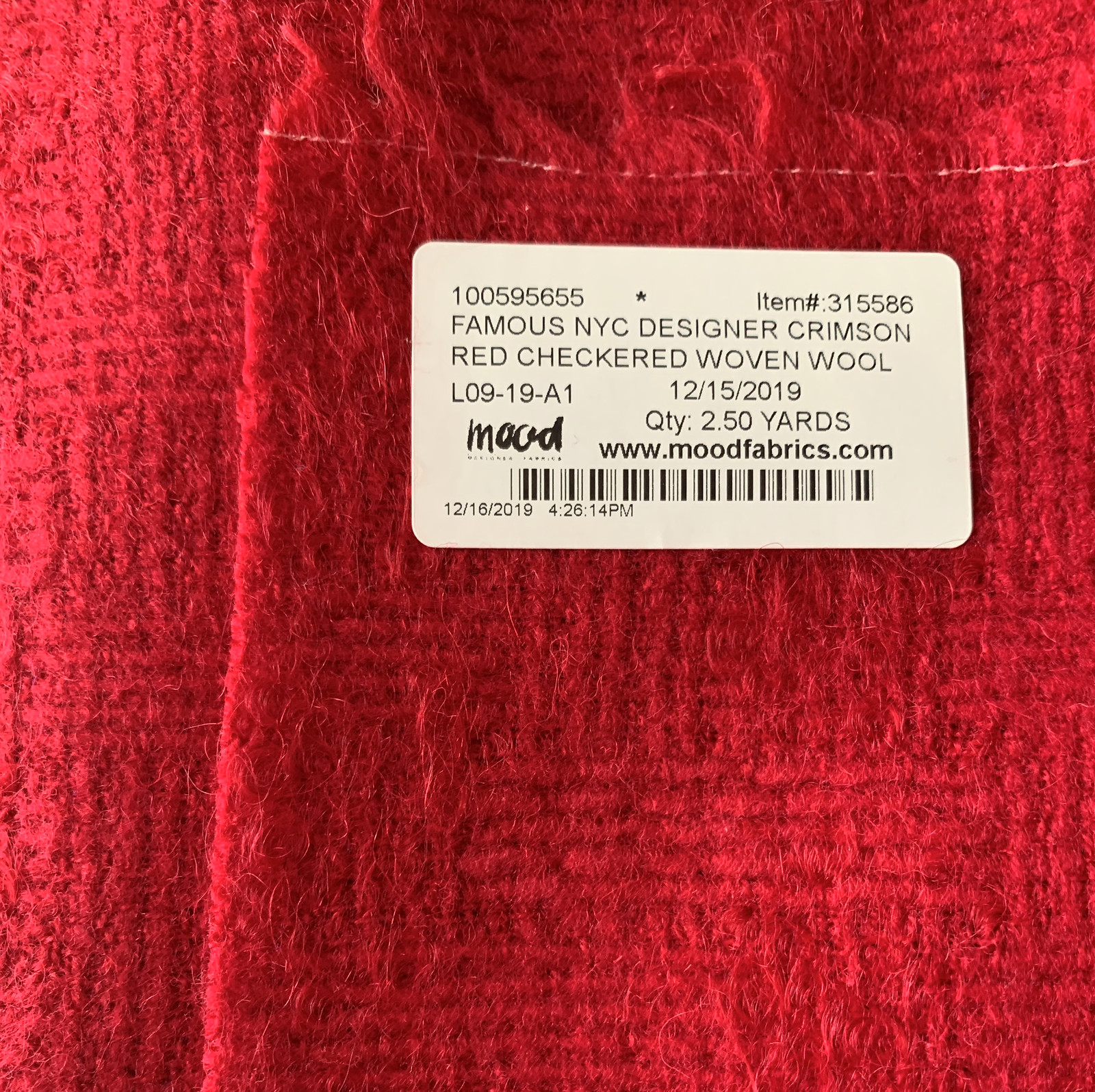This is an extremely close-up photograph of a bolt of crimson red checkered woven wool fabric, likely from a famous NYC designer. The fabric appears vibrant red, almost resembling a basket weave pattern. In the upper right quadrant of the image, there is a large rectangular white sticker occupying roughly a third of the photo. The bright white label, printed with black lettering, contains detailed information: "100595655, Item number 315586, Famous NYC designer crimson red checkered woven wool, L09-19-A1, 12/15/2019, Quantity 2.5 yards, www.moodfabrics.com." Below this text, there is a barcode, and in smaller print underneath, the date "12/16/2019, 2:26:14 PM." The sticker indicates that the fabric was bought from the website Mood Fabrics and provides specific item details and quantities.